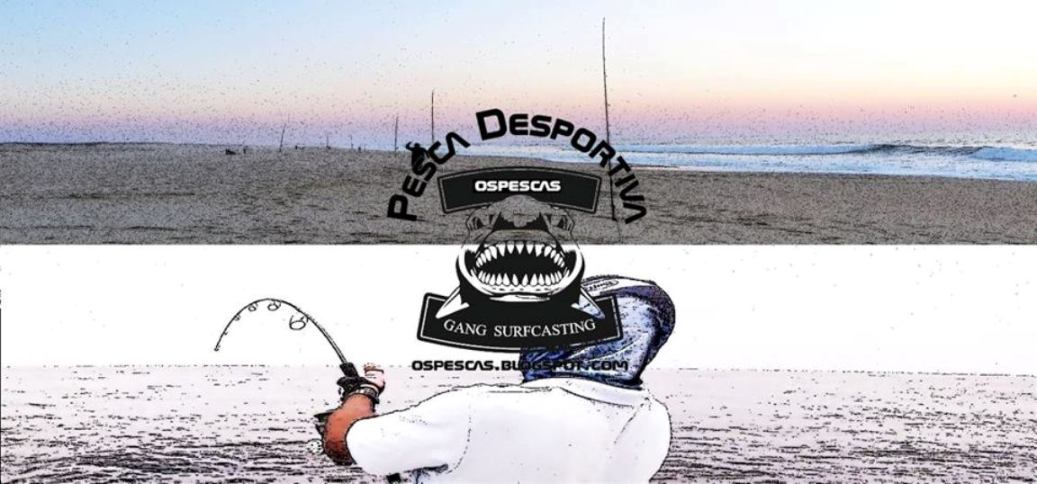In this composite advertisement image, we see two distinct sections stacked vertically, promoting a fishing event or activity. The top section showcases a serene beach scene with gentle waves crashing onto the shore and what appears to be fishing poles dotting the horizon. The colors in this upper part include shades of white, blue, and gray, capturing the tranquil seaside atmosphere.

The bottom section presents a dramatic close-up of an angler standing at the edge of a boat or pier, partially obscured by the composition. The angler, wearing a helmet-like device, is actively engaged in fishing, with a line visibly taut, indicating a catch. The colors here are more varied, including brown, purple tones.

Centrally positioned within the image is a prominent logo featuring a shark and the text "Pesca Desportum Aspectus Gang Surfcasting" or "Pesca de Sport AVM." The logo ties the two segments together, reinforcing the theme of sport fishing. This visual invitation, rich in dynamic detail and vivid color, seems expertly crafted for a collage or a fishing advertisement, effectively drawing the viewer’s attention to the excitement of the sport.